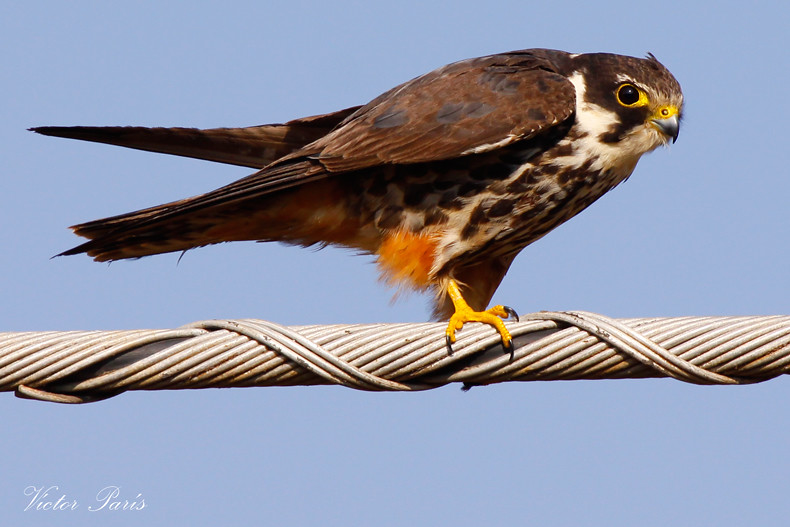This stunning close-up image, captured by professional photographer Victor Paris and signed in the lower left-hand corner, showcases a juvenile red-tailed hawk perched on a thick black electrical power cable wrapped in metal wiring. The background is a clear, light blue sky, emphasizing the bird’s striking features. The hawk is facing toward the camera with its dark eyes prominently seen. It exhibits a detailed feather pattern with brown and white splotches throughout its body. The bird's sharp black and white bill is topped with a yellow patch that extends above the bill and frames its eyes. The hawk's throat area is white, and its chest displays brown mottling. Its abdomen and tail area show hues of orange underneath, indicative of a red-tailed hawk, while the top of its head and wings are brown with darker brown splotches. Both wings are visible; the one closest to the viewer points downward to the left while the other points slightly upward. The bird’s yellow feet and sharp talons are clearly visible, gripping the wire securely, making it a captivating and detailed study of this majestic predator bird.